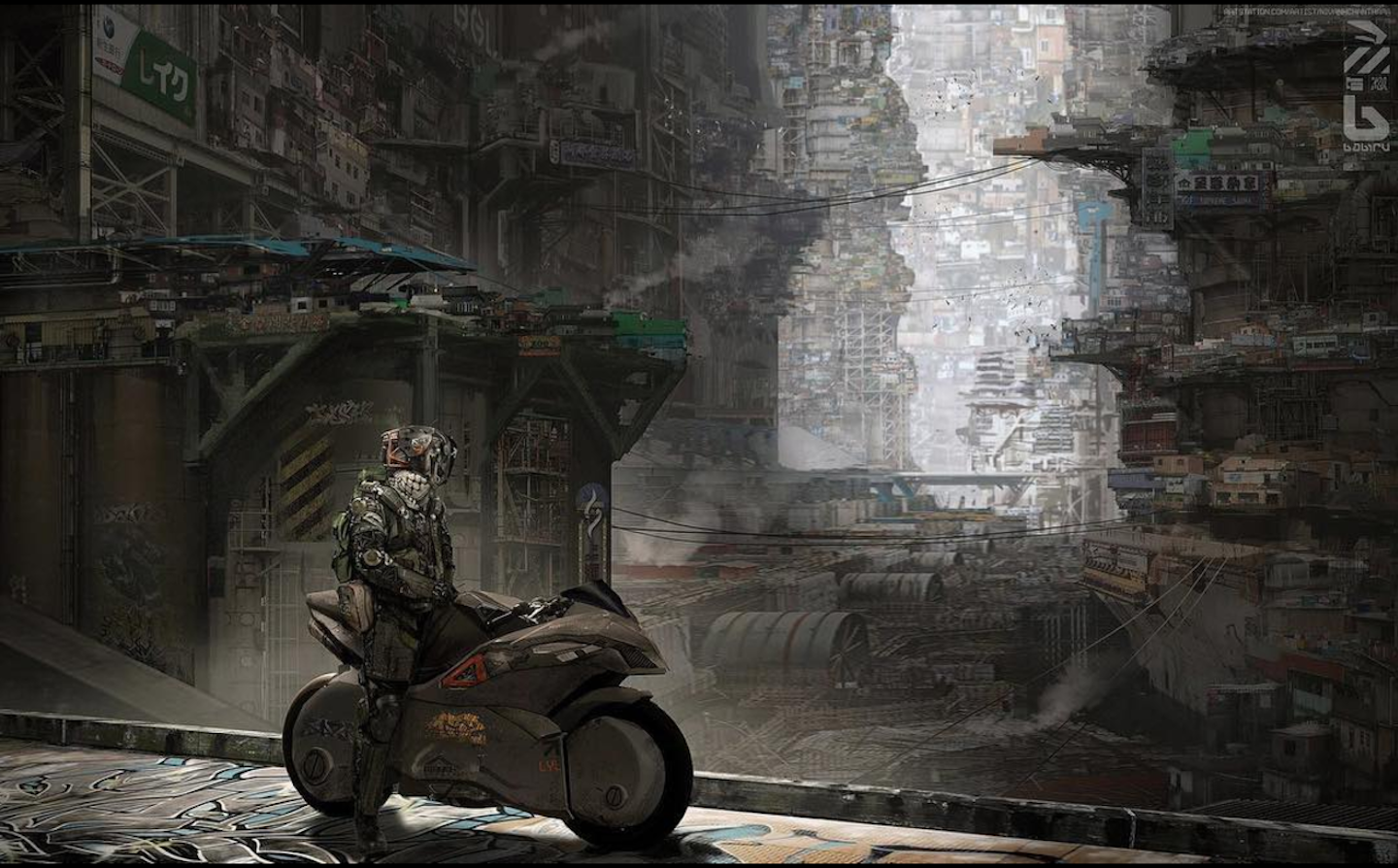The image depicts a dystopian, cyberpunk cityscape featuring a person on a futuristic motorcycle without a windshield. The rider, dressed in a black leather jacket and helmet obscuring their identity, is positioned in the bottom left of the frame, facing right and seemingly gazing into the horizon. The background reveals an array of tall, slender, glass and metal buildings emitting a bleak color palette dominated by dark gray, light gray, and black, with additional hues of beige, green, blue, tan, and silver. The scene is industrial and chaotic, showcasing metal barrels and graffiti scattered across an empty bridge. The streets below are deserted, further enhancing the desolate atmosphere. The overall feeling conveyed is one of isolation and a dystopian future.